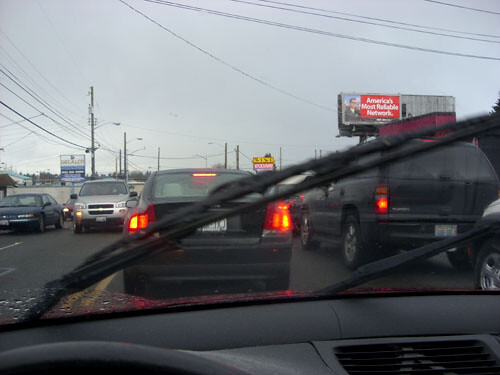A photograph captured from within a vehicle, equipped with a dashboard camera, reveals a scene of heavy traffic on a rainy day. The cloudy sky and wet windshield, onto which droplets are collecting at the bottom left and the wipers are positioned in the center, emphasize the ongoing rain. Multiple cars ahead, including a prominent black sedan immediately in front and a black SUV to the right, have their brake lights illuminated. On the left, a double yellow divider line separates the lanes with oncoming traffic, featuring a silver truck and a dark blue sedan among several vehicles. In the background, business signs and a billboard bearing the slogan "America's Most Reliable Network," accompanied by an image of a newscaster, are visible amidst the grey, overcast atmosphere. Power lines are also discernible in the distance.